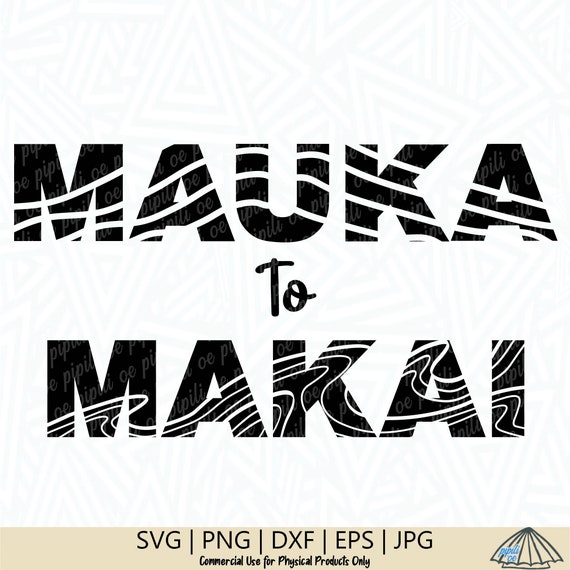The image displays a black and white graphic with a zebra-like or swirl pattern and features the text "Mauka to Makai" prominently. Beneath this text, a yellow banner lists the image formats: SVG, PNG, DXF, EPS, and JPG. Below this, a note states "commercial use for physical products only." To the right of the text, there is a simplistic black logo resembling an umbrella. There is also a watermark that is partially legible and might say "Piper."